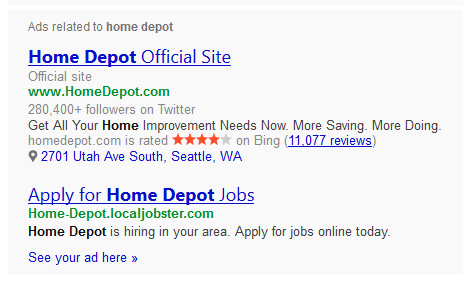This image is a screenshot of Google search results, specifically focusing on two advertisement entries related to Home Depot. The background is predominantly white. In the top left corner, there is text in thin, gray letters stating "Ad related to Home Depot", where "Home Depot" is displayed in bold, dark gray letters.

The first search result is labeled as the "Home Depot Official Site" in blue letters, with "Home Depot" in bold and underlined. Directly below this, the URL "www.homedepot.com" is displayed in green. Further down, it mentions "280,400+ followers on Twitter" along with a promotional blurb stating, "Get all your home improvement needs now; more saving, more doing," with the words "home improvement" in bold. Additionally, it notes that "homedepot.com is rated 4 out of 5 stars on Bing" from "11,077 reviews," and provides an address at "2701 Utah Ave South, Seattle, Washington."

The second advertisement reads "Apply for Home Depot Jobs" in blue letters, with "Home Depot" in bold. The URL "home-depot.localjobster.com" follows in green. The subtext beneath this heading says, "Home Depot is hiring in your area. Apply for jobs online today." Lastly, below this, there is a line encouraging advertisers with the text "See your ad here" accompanied by two right-pointing arrows, presented in blue.

The search results are tightly cropped, showing only these two entries without any additional web content.